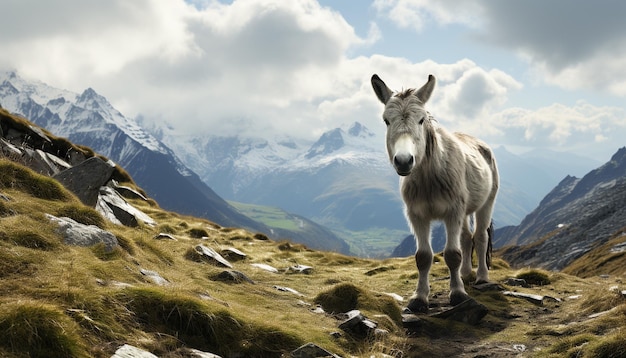The illustration captures a striking scene of a donkey standing regally on a sloping hill, which is situated to the right side of the frame. The donkey’s furry grey body possesses distinct features, including a white snout, a black nose, black eyes, and possibly a black tail. Its expression appears somewhat disinterested or sleepy, as it gazes directly at the camera. The landscape beneath the donkey's hooves is a patchwork of greenish-brown, unhealthy-looking grass with embedded grey rocks. 

In the distance, an impressive backdrop of blue-hued, snow-capped mountains stretches across the horizon, giving an impression of depth and serenity. Adding to the picturesque quality of the scene, the sky above is a vivid blue, dotted with large, fluffy white clouds, with a hint of grey in the top right corner. The overall outdoor setting harmoniously blends elements of animal life and natural landscape, creating a visually enchanting and richly detailed illustration.